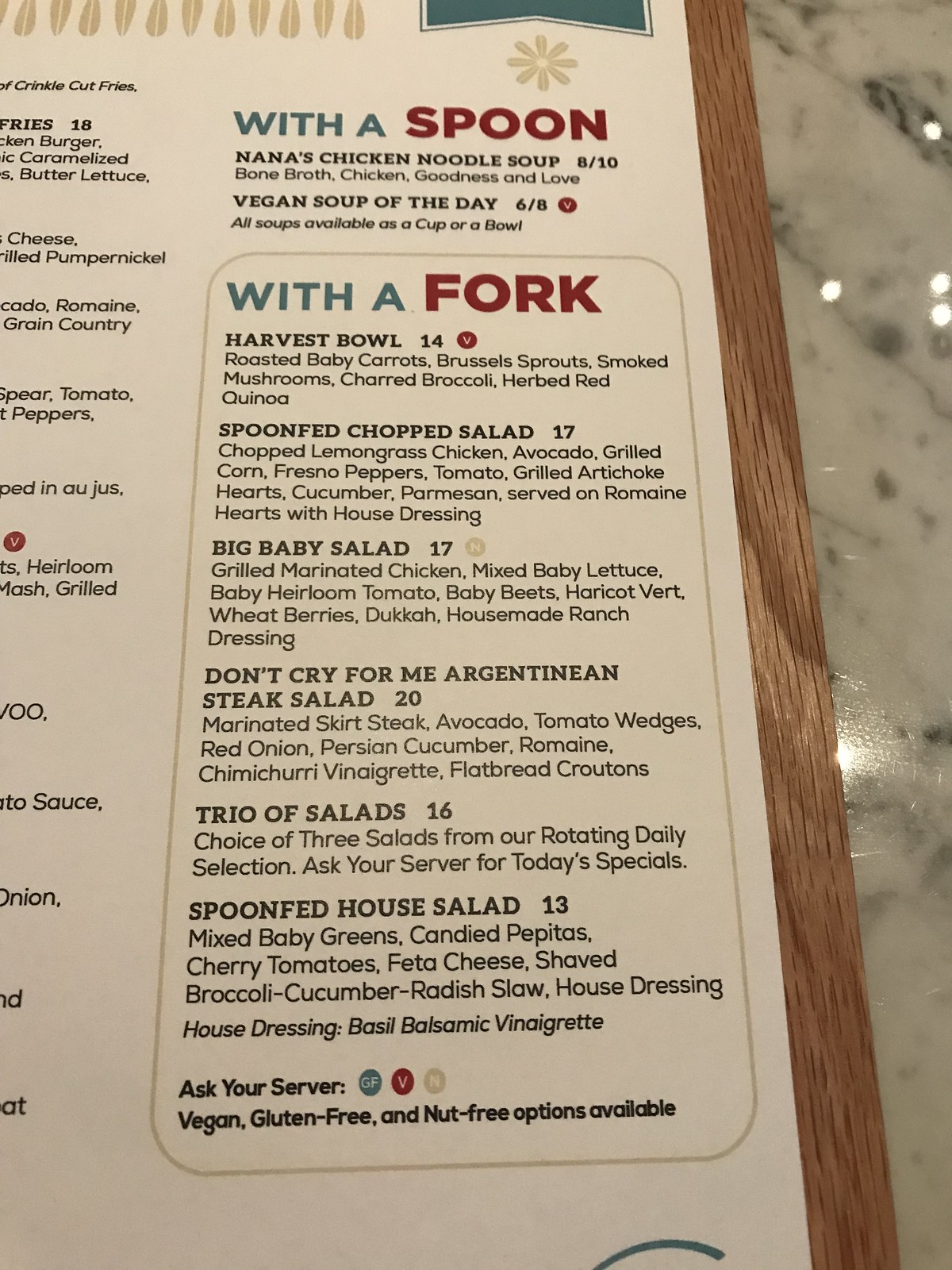The image depicts a detailed section of a restaurant menu, notably part of a sandwich and salad selection. The menu itself is presented on a sturdy material akin to a cutting board, giving it a robust and upscale appearance. It rests on what appears to be a glossy marble table.

The menu background is an elegant ivory color with black lettering, ensuring clarity and easy readability. To the far left, there are partial listings of sandwiches, with tantalizing ingredients such as fries, burger, lettuce, cheese, pumpernickel, and romaine, suggesting a diverse and appetizing selection.

Prominently featured in the middle section is a title labeled "WITH A SPOON," under which two items are listed: Lettuce Chicken Noodle Soup and Vegan Scoop of the Day. Below this, a section titled "WITH A FORK" lists an array of salads, each with its own unique name and description. These include:
- Harvest Bowl
- Spoon-Fed Chopped Salad
- Big Baby Salad ($17)
- Cross Me Argentina Steak Salad
- Trio Salad (Choice of Three Salads)
- Spoon-Fed House Salad

Each main dish title is in all capital letters, emphasizing the name, followed by a description in regular print. Particularly noteworthy is the variety of the salads, catering to different tastes and dietary requirements.

At the bottom of the salad section, a note advises customers to "Ask Your Server" about menu items, with icons indicating the availability of vegan, gluten-free, and nut-free options, ensuring dietary inclusivity.